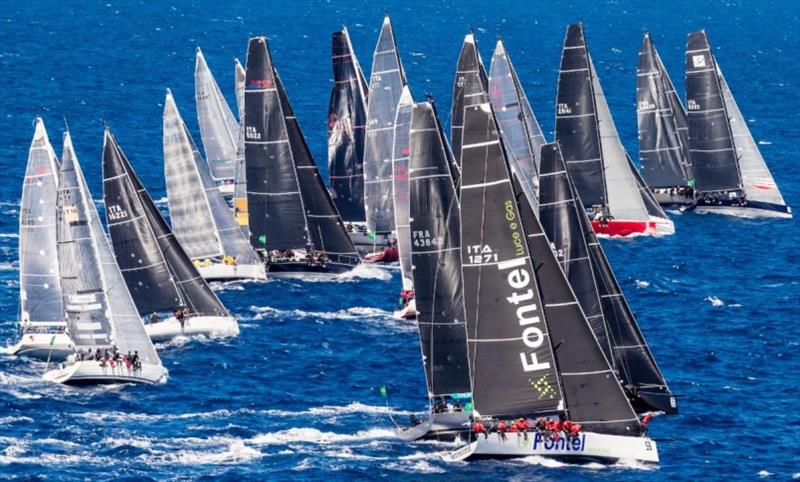This vibrant photograph captures a thrilling sailboat race in the deep blue ocean, characterized by its choppy, white-capped waves. Dominating the foreground is a sleek white sailboat with the name "FONTEL" emblazoned in bold blue letters on its side and again in white letters on its towering black sail, which also displays "ITA1271." The boat is teeming with crew members clad in striking orangey-red jackets, poised for action. Surrounding this focal boat are approximately 15 to 20 other sailboats, clustered closely in the water, some of which appear nearly to touch each other as they lean in unison, propelled by a strong wind. The majority of these boats feature black sails, though a few display silver, white, or even transparent sails, adding dynamic contrast. Most hulls are white; however, there's a distinct red sailboat with a black sail, enhancing the colorful array. Sunlight gleams off the sails, illuminating the scene with a bright, sunny glow, suggesting a clear day full of intense competition and vivid scenery.